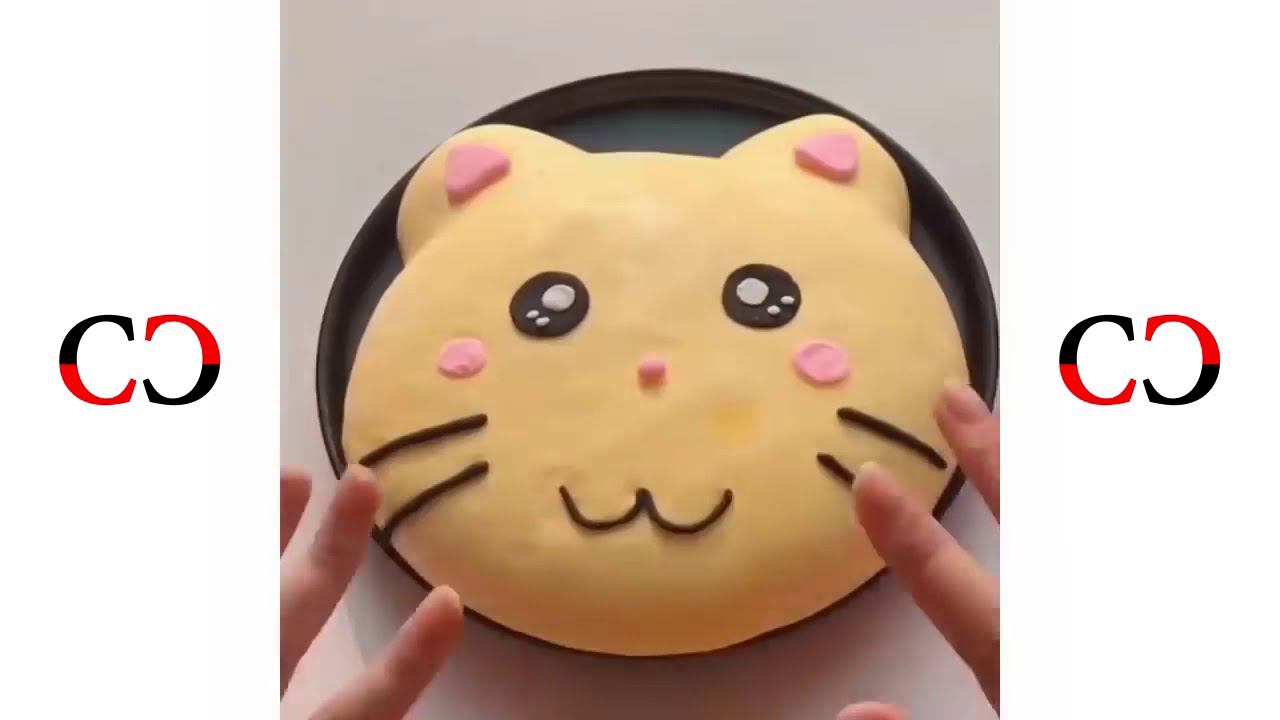In an off-white background, an animated cat-like creature sits in a round cake pan made of sheet metal, resembling a large cookie or pastry. The creature has light yellow or light orange frosting with pink tips and centers on its ears, rosy cheeks, and a pink nose. Its black eyes glisten with three white dots in each, accompanied by two black whiskers on either side of its W-shaped mouth. On the left and right edges of the image, there are vertical white bars featuring a logo with the letters "CC," where the forward-facing "C" is mirrored with a backwards "C." Each "CC" logo is split into red and black colors. The bottom of the image shows the fingertips of a person on either side of the cake.